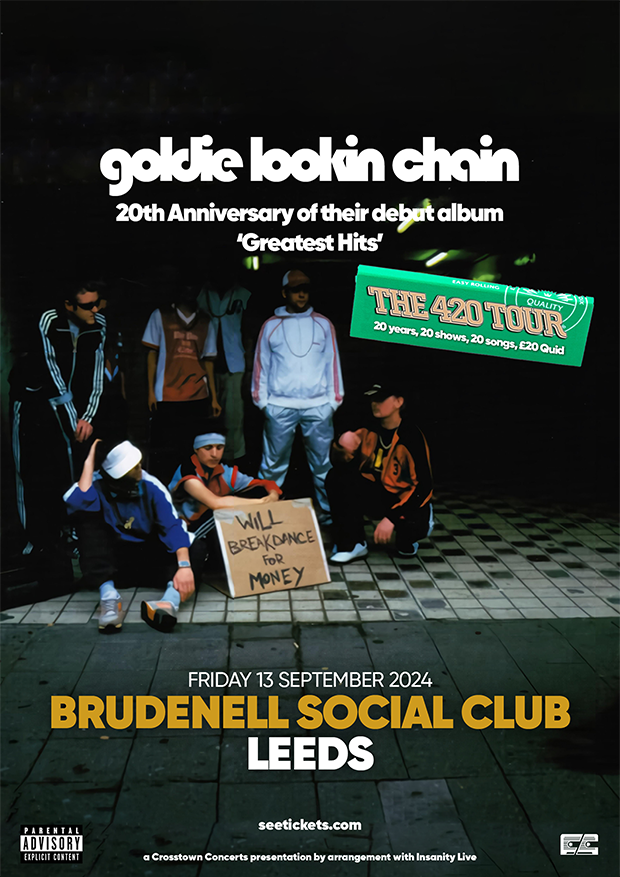The image showcases a vibrant, color photograph made to resemble a poster for an event. The backdrop is predominantly black, creating a striking contrast with a group of people dressed in modern retro streetwear, including Adidas tracksuits and hoodies. They pose on a black and white tiled floor, resembling a street scene. Some individuals are standing while others are seated, adding depth to the composition.

A notable detail is a brown cardboard sign placed amongst the group, which reads "We'll break dance for money" in bold black ink, delivering a gritty, earnest vibe. At the top of the image, bold white text announces, "Goldie Lookin' Chain, 20th Anniversary of their debut album, Greatest Hits". The central text reiterates this anniversary with the 420 Tour's taglines in orange, "20 years, 20 shows, 20 songs, 20 quid."

At the bottom, details of the event are displayed: "Friday, 13th September 2024, Brudenell Social Club, Leeds," alongside a website for tickets. The image is flanked by iconic symbols – a Parental Advisory label in the bottom left corner and a cassette icon in the bottom right. Collectively, these elements evoke a sense of nostalgia mixed with contemporary flair, celebrating the legacy of Goldie Lookin' Chain while grounded in the urban culture of breakdancing.